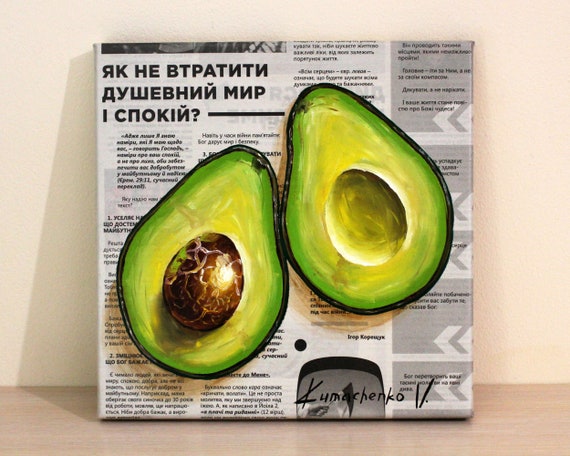This artwork is a mixed-medium piece, square in shape, leaning against a beige wall, and situated on a wooden surface or floor. The canvas appears to be made from newspaper, tightly wrapped around a flat board, giving it a beveled effect. The newspaper is in a Slavic language, featuring a mix of black and white text with some grayed-out sections. At the center of the canvas, two ripe avocado halves are painted. The left half contains a large brown pit, while the right half has an empty pit indentation. Both halves display a light green interior with darker green edges, and the skin is thin and black. The detailed composition blends the textured look of the newspaper with the vivid colors of the avocado, creating a striking visual contrast.